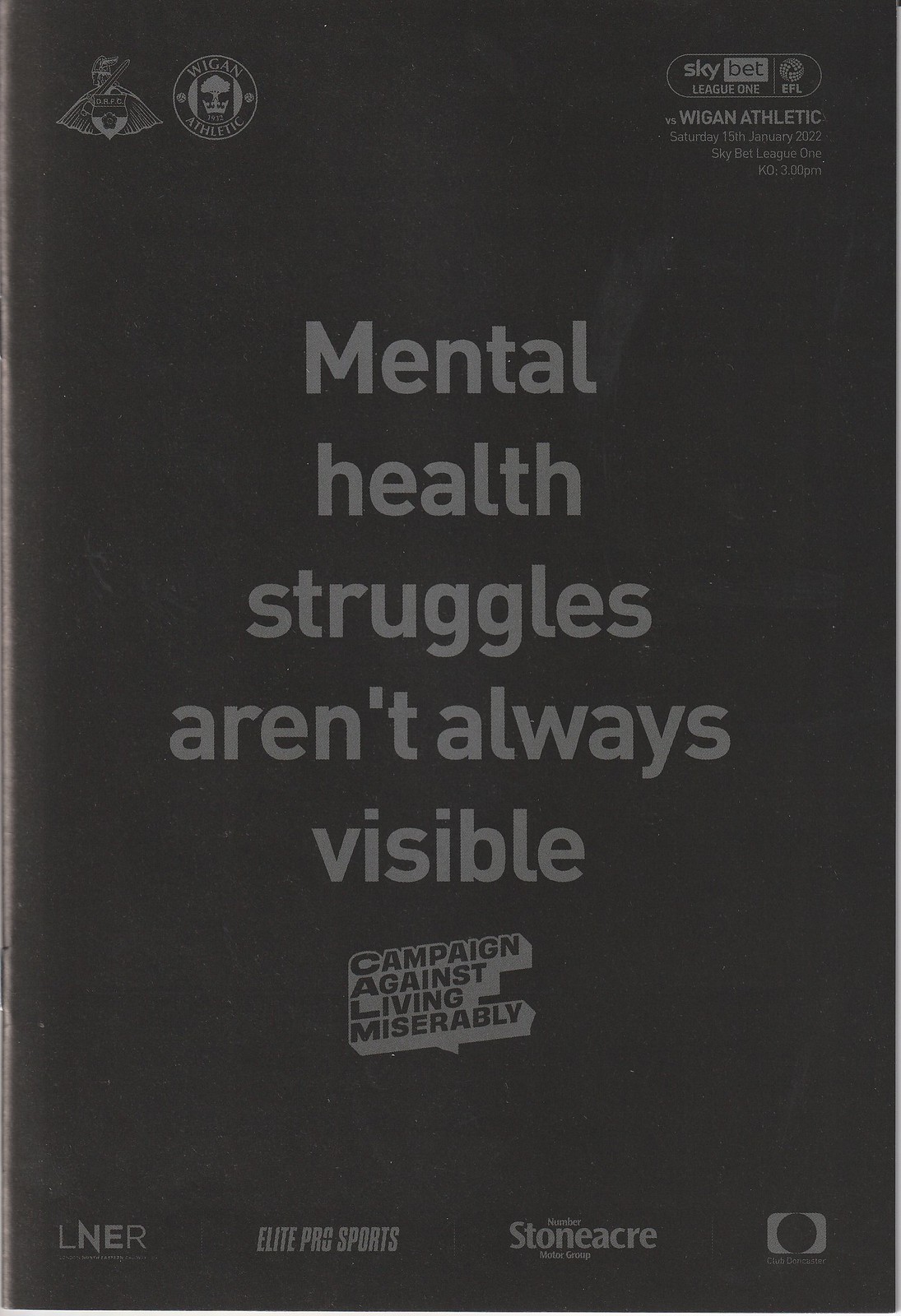The image depicts a dark, monochromatic flyer or poster with a black background and dark gray text, creating a somber and serious tone. At the top of the flyer, there are icons representing sports teams, including one that features a crest resembling a Viking with a sword and shield, symbolizing a soccer team, and another emblem for Wigan Athletic. To the top right, text indicates an upcoming match: "versus Wigan Athletic, Saturday, 29th January 2022". The main message of the poster, prominently centered, reads, "Mental Health Struggles Aren't Always Visible." Below this poignant statement, a logo appears for the organization "Campaign Against Living Miserably," emphasizing the cause. The lower section of the flyer showcases a row of sponsor logos, including entities like Liner, Elite Pro Sports, Stoneacre, and a distinctive 'O' logo, among others. There is also the Sky Bet League One EFL logo at the top right. The overall design suggests a connection between the sports event and a broader mental health awareness campaign.